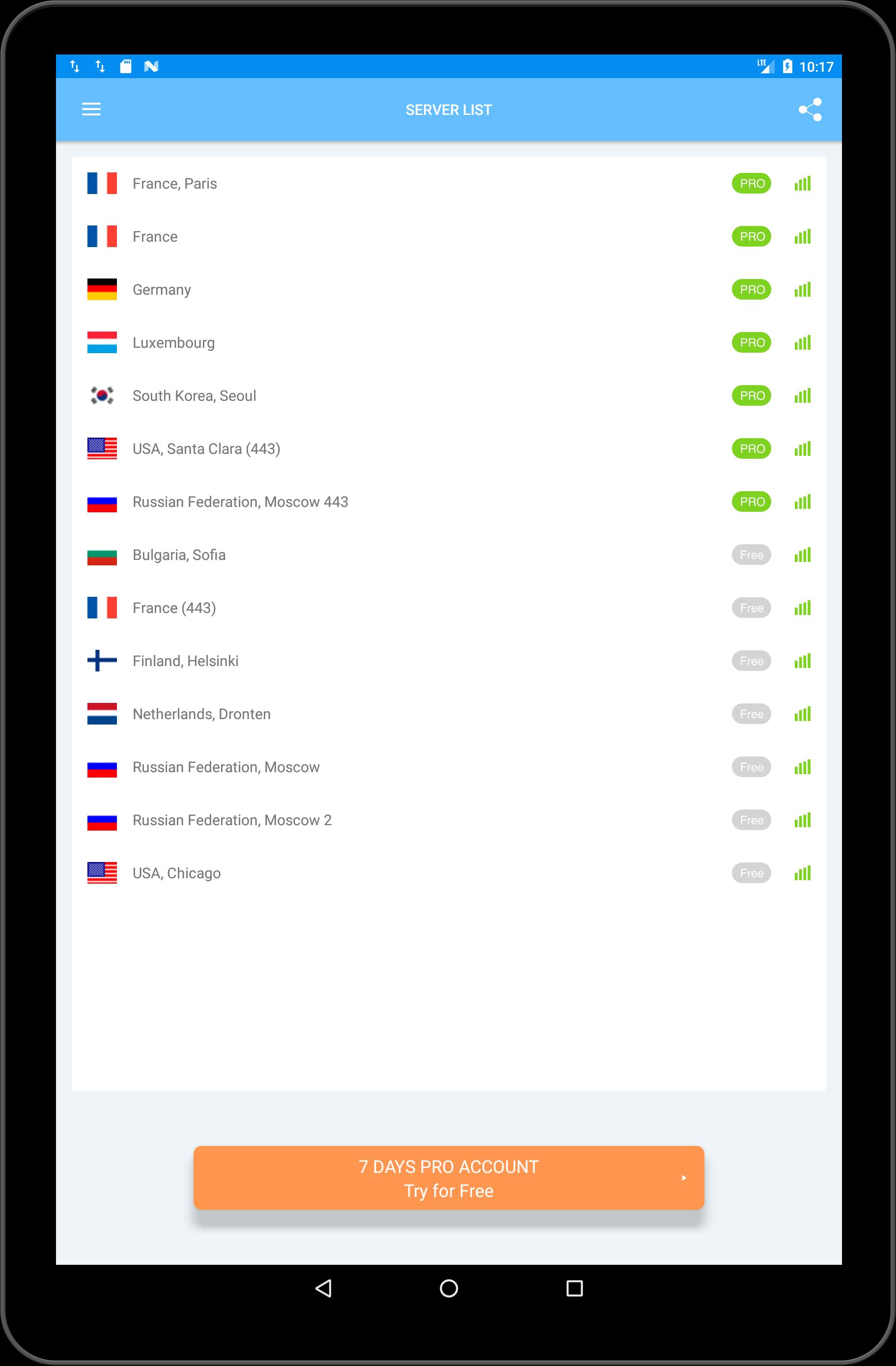This image is a screenshot of a tablet displaying a server list interface. At the top, there's a blue navigation bar with the label "Server List." On the left-hand side of this bar, there are three horizontal lines, suggesting a dropdown menu. On the right-hand side, there are three vertically connected dots, whose purpose is unclear.

The main section of the screen features a white background where a list of servers is displayed. Each server entry includes the country, city, and sometimes specific identifiers such as port numbers in parentheses. Here is the list:
- France, Paris
- France
- Germany
- Luxembourg
- South Korea, Seoul
- USA, Santa Clara (443)
- Russian Federation, Moscow (443)
- Bulgaria, Sofia
- France (443)
- Finland, Helsinki
- Netherlands, Dronten
- Russian Federation, Moscow
- Russian Federation, Moscow 2
- USA, Chicago

To the right of each server entry, there are labels indicating whether the server is free or requires a pro-level subscription. The first six or seven entries are marked as pro-level, while the rest are labeled as free.

Adjacent to these labels are signal strength bars, likely representing the quality or speed of the connection. Each server entry also features the corresponding national flag to the left. For instance, the server entry for Paris, France, is accompanied by the French flag.